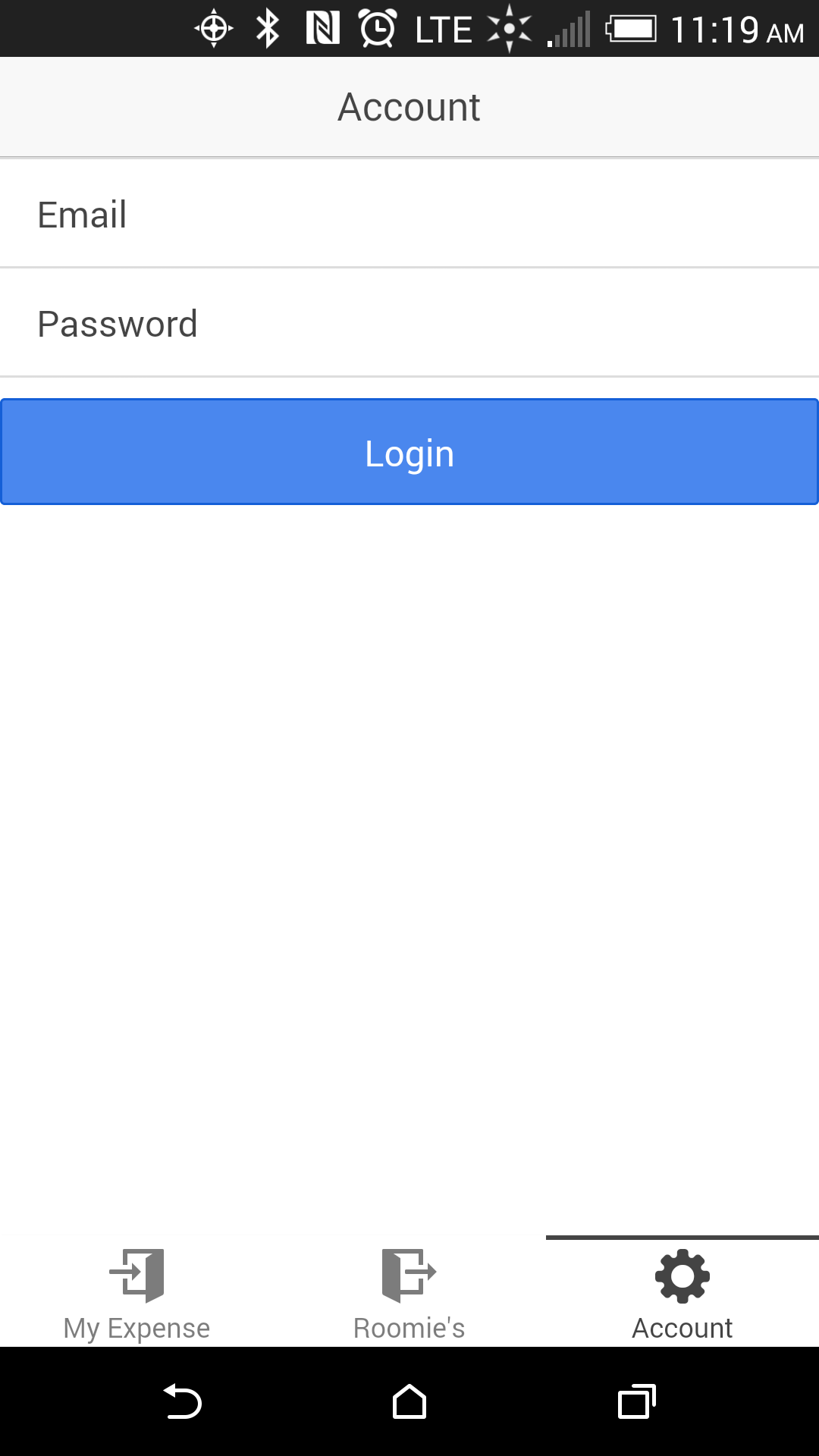This is a detailed screenshot seemingly taken from a phone, likely an Android device. At the top of the screenshot, there's a black status bar featuring several icons. Starting from the left, there's an icon resembling a target, followed by a Bluetooth icon. Next to these is an icon that looks like an "N" within a square. This is followed by a clock icon alongside an LTE symbol. There's also an icon that looks like a sun, depicted as a dot with small triangles around it, and a signal bar icon showing just one bar lit, indicating weak signal strength. Adjacent to this is a fully filled battery icon and a timestamp reading 11:19 AM.

Below the status bar, in a light gray area, it reads "Account" under the heading "Flush Center." Directly beneath this, there are fields labeled "Email" and "Password." Below these fields, there is a long blue rectangle button centered on the screen labeled "Login."

The middle section of the screenshot is blank and white. Near the bottom, on the left-hand side, it says "My Expense" with an icon that looks like a door with an arrow pointing to the right. Next to this, it says "Roomies" alongside another door icon with an arrow pointing to the right, but the door is depicted in the opposite direction. Lastly, it says "Account" next to a cog icon with an arrow and an underscore symbol placed above it.